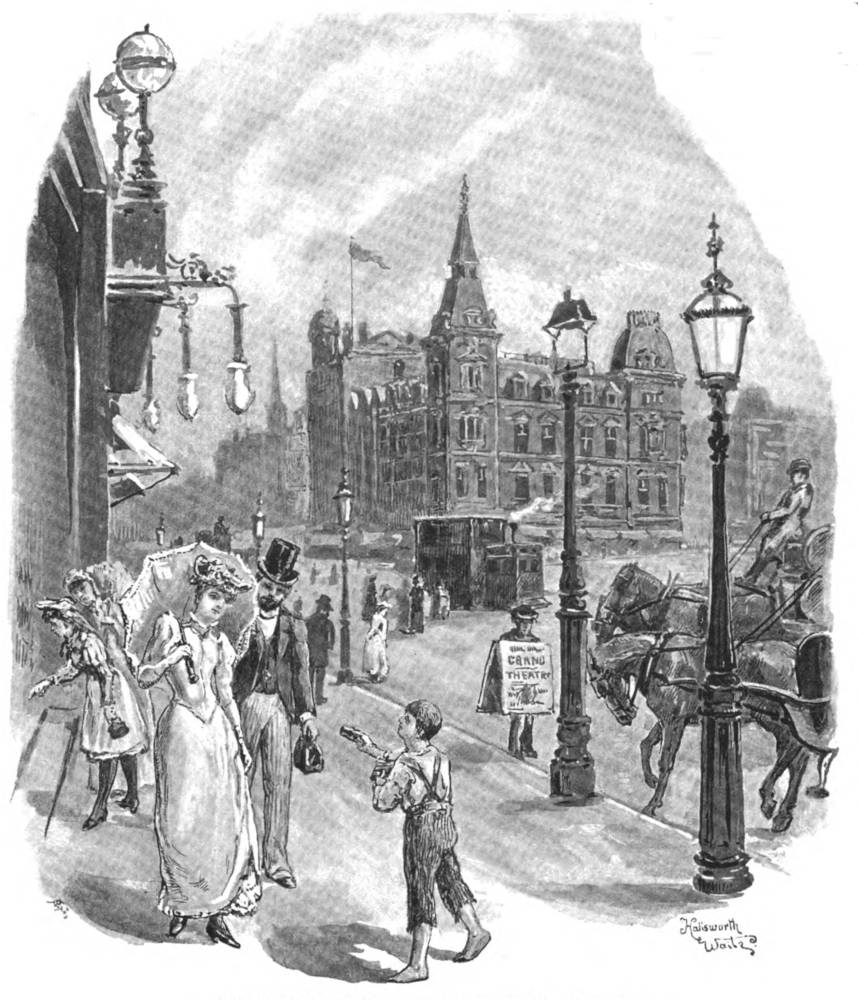This detailed black-and-white pencil sketch illustrates a bustling city street from a bygone era. On the right side, horses are tethered near lamp posts, setting a historic ambiance. In the lower center, a well-dressed man in a top hat and suit stands beside a woman in a dress holding an umbrella. A young boy in overalls extends his hand towards them, perhaps begging or attempting to sell something. The scene is imbued with themes of class disparity, contrasting the refined attire of the couple with the boy's humble appearance. In the background, buildings with pointed spires rise above the street, while streetlights line the sidewalk, emphasizing the busy urban setting. There is also a person wearing a sandwich board sign, adding to the street's vibrant narrative. The artist has signed the piece in the bottom right-hand corner, completing this evocative portrayal of social contrasts in an antiquated cityscape.